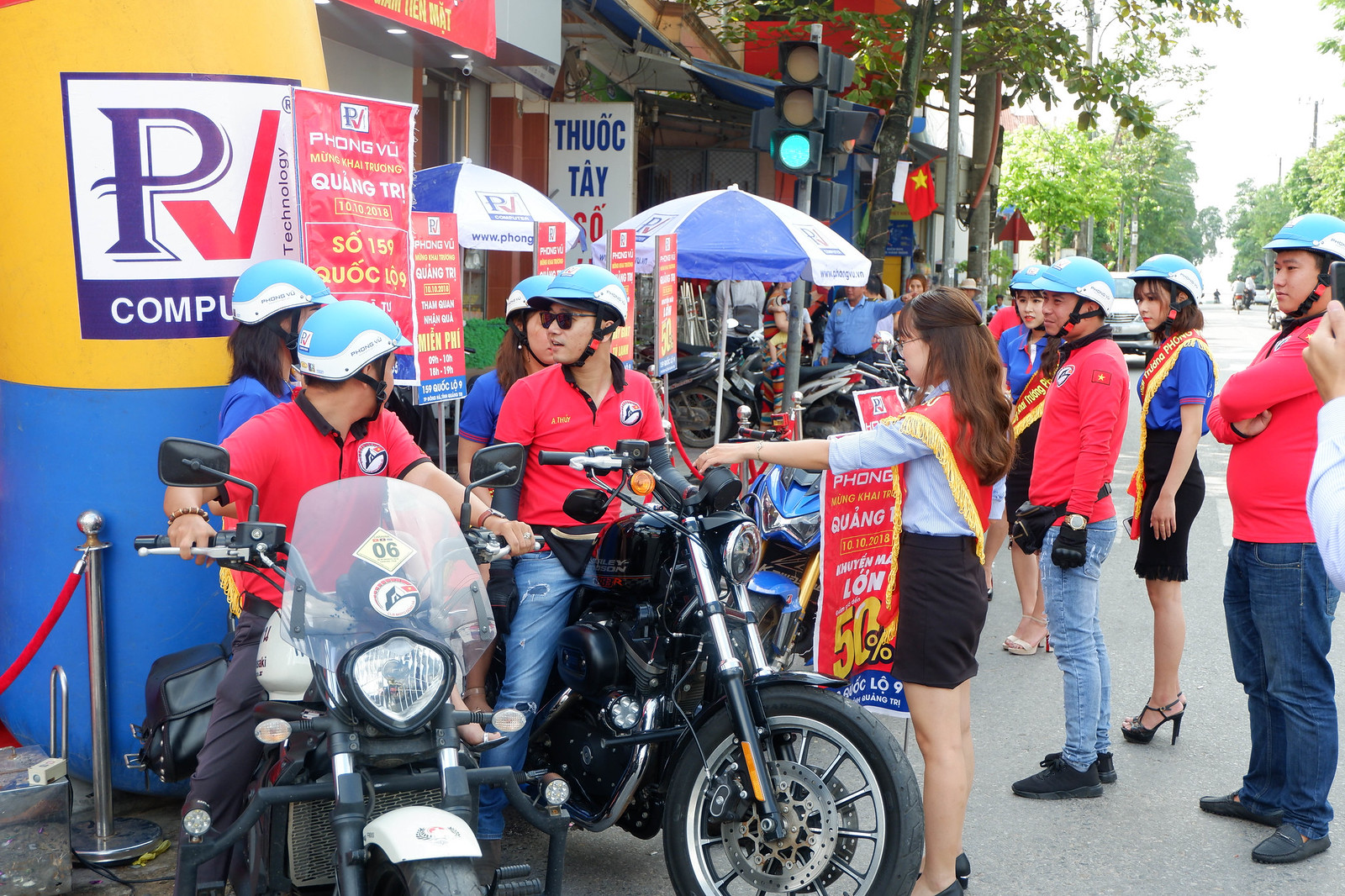This photograph captures a vibrant scene set in what appears to be an Asian country, possibly Vietnam. It features a group of people, some standing and others astride motorcycles, all gathered on a busy street. The individuals on the motorcycles and several of the standing participants are uniformly dressed in red shirts, blue pants, and blue and white helmets, suggesting they are part of a motorcycle race or group. Among them is a woman distinguished by her safety vest and black skirt, standing in front of one of the motorcycles. She has brown hair and is notable for coordinating or supervising the activity.

In the background, there's a strip of buildings along with green trees and a white sky. Outdoor café-style seating is evident, with tables sheltered by blue and white umbrellas, enhancing the vibrant, communal atmosphere. A noteworthy feature is a large blue and yellow cylindrical balloon or banner on the left side of the image, bearing the incomplete text "PV technology" with a checkmark-like "V" and additional wording, possibly "computers," partially obscured.

Additional signs and banners in the vicinity, including one reading "Fong Vu Quang Tri," contribute to the locale's bustling ambiance. The crowd also includes individuals in black skirts with yellow and red sashes over their shirts, adding to the varied and colorful attire seen throughout the gathering. The meticulous array of coordinated clothing and equipment underscores the organized nature of the event, making the scene both dynamic and picturesque.